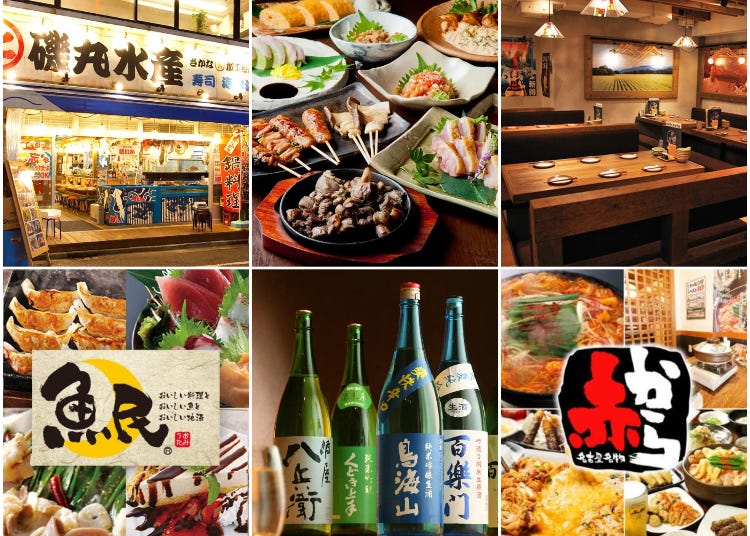The image is a rectangular collage composed of six square photographs separated by thin white lines, showcasing various aspects of a Japanese restaurant. In the top left, a photograph depicts the restaurant's storefront adorned with a large sign featuring black Asian characters, accompanied by red banners and signboards. The top middle image focuses on an array of seafood and meat dishes displayed on plates, including beef bowls, skewers, and a variety of bowls in different materials. To the top right, there is a booth seating area with a horizontal rectangular table set with six plates and chopsticks, featuring dim lighting, backrests, and wall-hung pictures.

The bottom row begins with the left image showing several food items such as cheesecake and gyoza presented on plates. The bottom center image features four bottles of alcoholic beverages, likely sake, with two bottles tinted blue and the other two green, each adorned with labels in various colors and scripts. Finally, the bottom right image revisits the theme of multiple dishes, including hot pot and additional booth seating depicted in a smaller collage format. Throughout the images, elements like Japanese writing, a crescent moon logo, and a mixture of traditional and modern dining aesthetics contribute to an authentic dining experience portrayal.